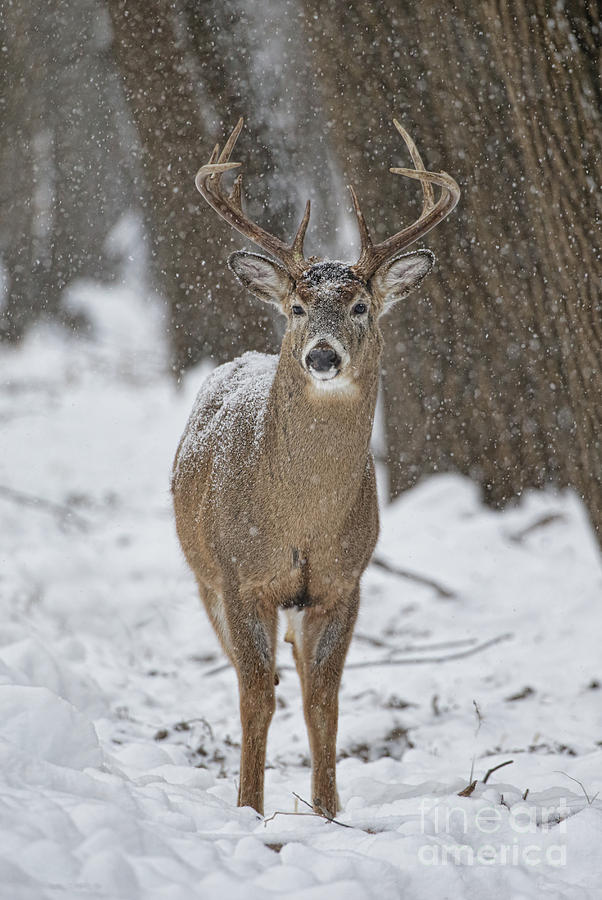The image is a vertically aligned rectangular picture featuring a brown buck standing in a snowy forest, staring directly at the camera. The ground is thickly blanketed in white snow, visibly disturbed with numerous footprints. Snow is falling from the sky, creating a serene atmosphere. Brown grass and sticks poke out from the snow near where the deer is standing. The deer has dark brown fur with white on top and around its mouth, a black nose, and tan colored ears with dark outlines. Snow has landed on its back, head, and antlers. The antlers, two on each side, curve inward. In the background, several large tree trunks are visible but become increasingly blurry, particularly a very large one in the upper right corner. The image, marked with "Fine Art America" in the corner, has an appreciation for nature that draws the viewer into the serene, wintry scene.